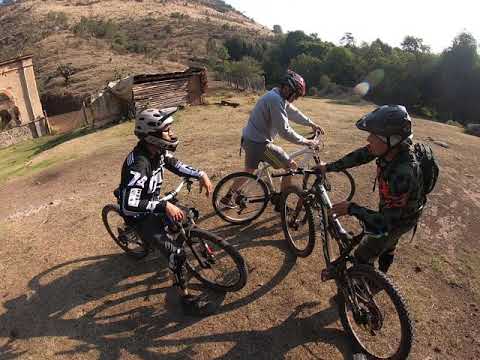This photograph captures three men on bicycles in a remote, hilly area with a rustic ambiance. They appear to be in conversation, gathered on a dirt clearing surrounded by natural elements. The backdrop features a dense concentration of trees on the right, with a prominent mountain or larger hill that extends upward to the upper left corner of the image. An earthy hut, partially visible, nestles into the landscape with green grass and brown stones in front.

In the foreground, the man on the left is outfitted in a distinctive black racing uniform marked with the number 74 and a BMX helmet. He is seated on his bike, which has black and red accents, and is attentively looking to the right. At the center, another man is balancing with one foot on a bike pedal, wearing brown shorts, a gray shirt, and a helmet with red markings, appearing engaged with the others. The third man on the right is standing beside his bike, dressed in a black outfit with red details on the chest, a dark helmet, a backpack, and facing the left toward his companions.

The sun casts shadows on the ground, emphasizing the brightness of the day and the clarity of the scene. Despite the rustic setting, the men’s attire and equipment suggest they are here for a purposeful biking excursion, pausing perhaps to discuss their route or enjoy a moment of camaraderie amidst the serene, untamed backdrop.